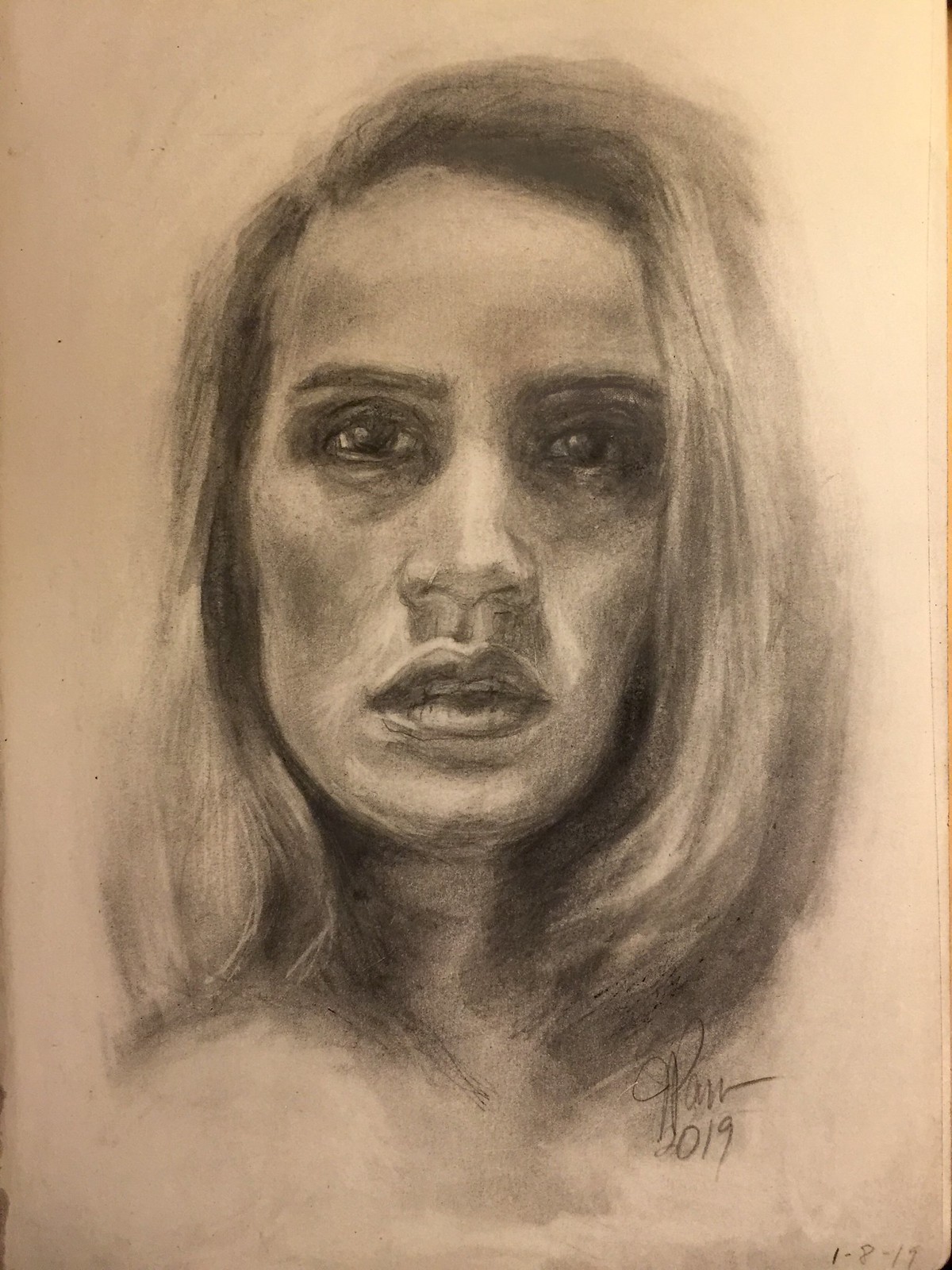This captivating charcoal drawing depicts an intensely focused woman seen from the neck up, created on textured white sketch paper. The close-up portrait captures her steady gaze with large, dark eyes that seem to peer directly into the viewer's soul. Her expression is neutral, with her slightly parted lips subtly revealing her teeth. Her long, straight hair is parted to one side and cascades down to about shoulder length. The intricate detailing in the drawing underscores the artist's skill in rendering lifelike features with charcoal. In the bottom right-hand corner, the artist has signed the work and included the year "2019," indicating the piece's creation date.